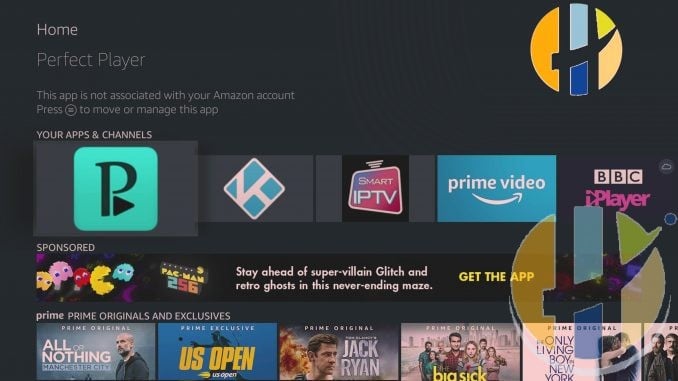This screen capture showcases a user interface with a gray background. At the top of the image is a navigation bar featuring the text "Home" and "Perfect Player," both in gray. A message indicates that the app is not associated with the user's Amazon account. There is an icon button labeled with instructions to move or manage the app.

In the upper right corner of the screen, there is a multi-colored circle containing segments of orange, blue, and green. Beneath this, the interface displays a category titled "Your Apps and Channels," presenting several icons in a row: a turquoise and black icon, a light blue and white one, a pink and white one, a blue and white icon labeled "Prime Video," and a pink and white icon for BBC iPlayer.

Further down, a section labeled "Sponsored" displays a promotional banner for the game Pac-Man 256, featuring gold, pink, red, and blue Pac-Man characters. The description reads, "Stay ahead of supervillain glitch and retro ghost in this never-ending maze." A yellow button invites the user to "Get the App," accompanied by the previously mentioned multi-colored circle icon.

Continuing down the page, another section is labeled "Prime Originals and Exclusives." It showcases several titles with accompanying images: 
1. "All or Nothing Manchester City" with a blue background and a man.
2. "US Open" displaying a tennis player in action.
3. "Jack Ryan," featuring a man with brown hair against a backdrop of an explosion.
4. "The Big Sick," showing various people with a city skyline in the background.
5. "The Only Living Boy in New York," with a picture of people hugging.
Below this, partially visible, is an image of several men.

The layout and organization of the content provide a comprehensive overview of available apps, sponsored content, and exclusive Prime offerings.